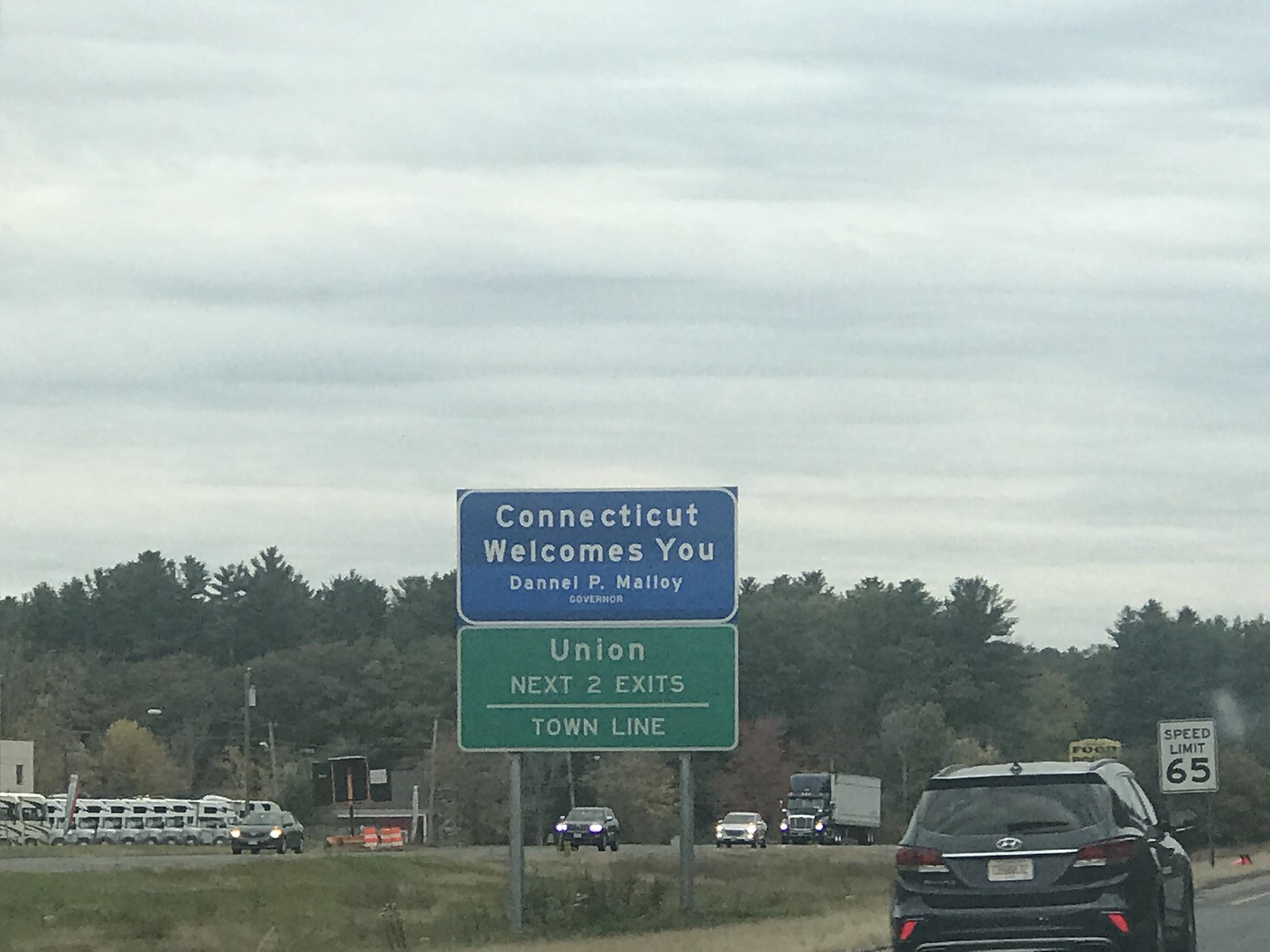A photograph captures a two-way road bordered by a dense forest of evergreen trees in the background. The road features two lanes of traffic heading away from the viewer and two lanes coming toward, separated by a grassy ditch-like median. The oncoming vehicles have their headlights on, illuminating the scene. Prominently displayed along the road are various signs: a speed limit sign indicating 65 mph, a blue rectangular sign welcoming travelers to Connecticut with the message, "Connecticut welcomes you, Dan L.P. Malloy, Governor," and a green rectangular sign announcing, "Union, Next Two Exits, Town Line." The lush green grass in the median adds a touch of natural beauty to the bustling roadway.